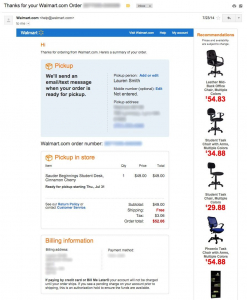**Caption:**

The image features a primarily white background with various elements scattered across it. At the top, there is a small white square containing the text "Thanks for your Walmart.com order," followed by some blurred-out information. Below this, there is a small yellow spot next to a tiny blue box that includes very small, unreadable print and what appears to be a blue search box.

Further down on the white background, there is a prominent blue box with the word "PICKUP" in red letters, accompanied by a specified time, partially blurred. Beneath this, a thin blue line separates it from another blue-outlined box, inside which a red package icon is visible with the text "Pickup in store" beside it. The same box displays prices in both blue and red colors.

At the bottom, there is a final box labeled "Billing Information," but all the specific details in this section are blocked out. On the right-hand side of the image, there are several product recommendations featuring different office chairs with their prices listed as $54.83, $34.88, $29.80, and $54.88.